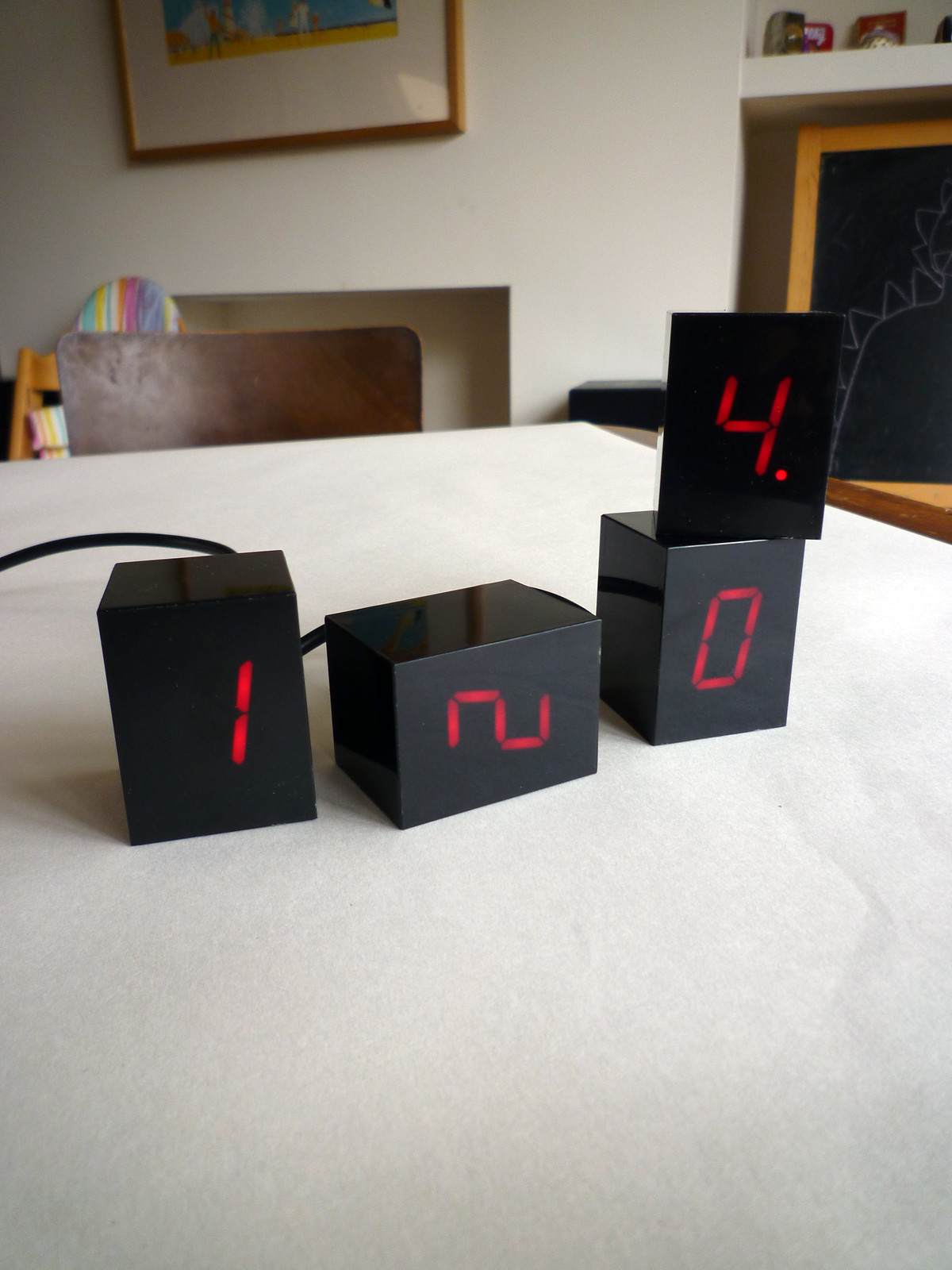The photograph showcases four black plastic boxes, each displaying a single-digit red LED number. The boxes appear interconnected through an electrical cord extending out of the frame to the right. The setup rests on a white table covered with a slightly wrinkled paper or cloth, hinting at imperfections on the surface. From left to right, the first box features the number "1," the second box is positioned on its side showing the number "2," the third block displays a "0," and the fourth block, positioned atop the previous one, shows "4" followed by a decimal point.